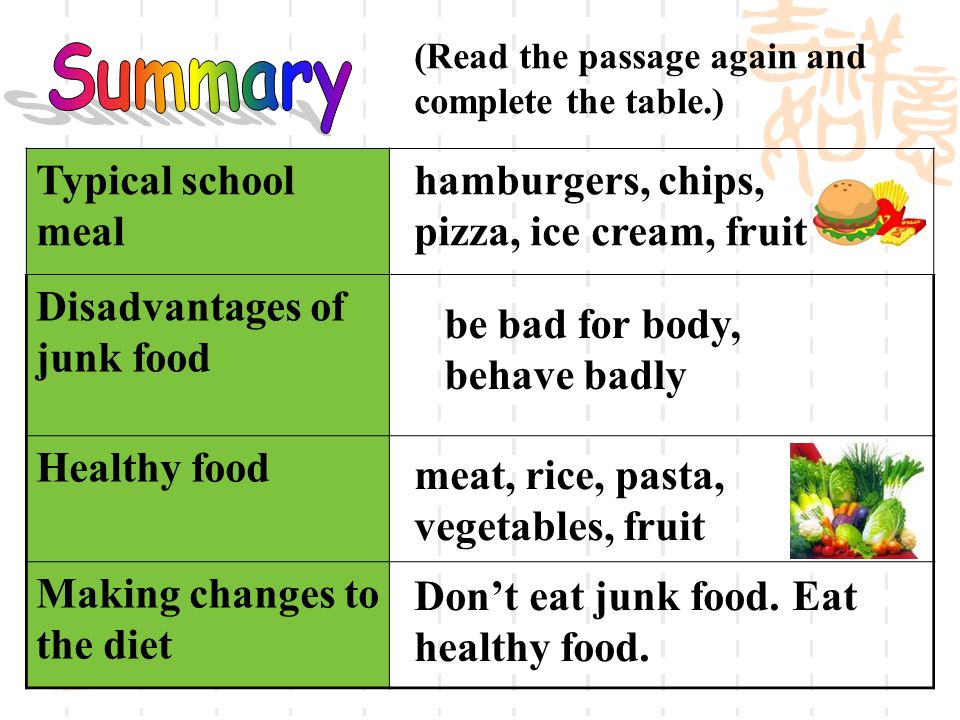The image depicts an informational poster likely intended for a school setting, with a clean white background. In the upper left corner, the word "summary" is vividly displayed in rainbow-colored letters with gray shading, giving it a 3D effect. To the right of this, in black letters enclosed in parentheses, it instructs "read the passage again and complete the table." Below this, on the left side, there are four green rectangular segments with black text, each corresponding to white rectangles on the right side containing further details.

The first green segment is labeled "typical school meal" and to the right, in the corresponding white rectangle, it lists "hamburgers, chips, pizza, ice cream, fruit," accompanied by a computerized image of a hamburger and fries. The second segment, labeled "disadvantages of junk food," describes in black text "be bad for body, behave badly." The third segment titled "healthy food" lists "meat, rice, pasta, vegetables, fruits" with an associated image of these food items. The final green segment, "making changes to the diet," advises "don't eat junk food, eat healthy food." 

In the upper right corner of the poster, there are faint, tan-colored Asian symbols. This stylistic choice, along with the computerized images and straightforward text, suggests the poster is a structured, educational tool designed to inform children about nutrition and dietary choices.